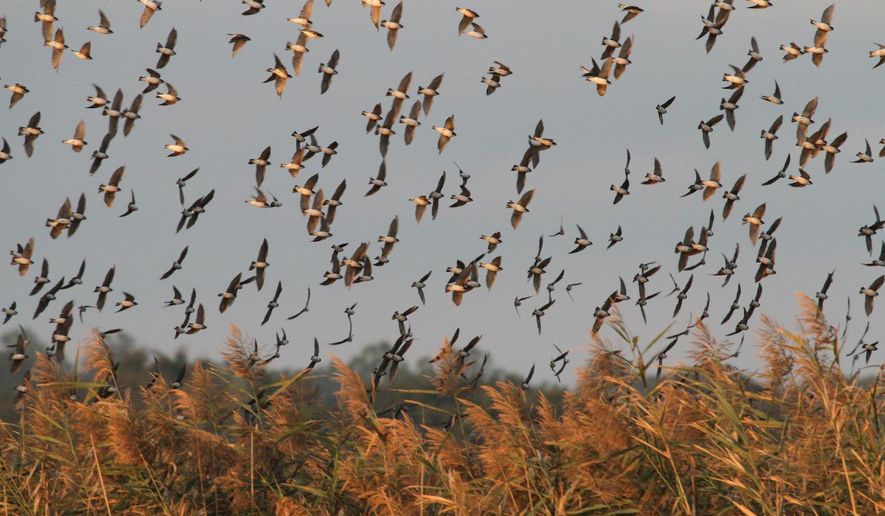In this captivating nature photograph, a sizable flock of small birds is captured in mid-flight. These birds, characterized by their white bellies and black and brown wings, are depicted against a serene, clear grayish-blue sky devoid of clouds. The birds, numbering between 50 to 100, are flying in various directions, with most heading from right to left. Their wings are outstretched, likely caught in the midst of beating.

Beneath the birds, a field of wild, orange-brown and green brush stretches out, resembling tall grasses or wheat swaying gently in the wind. The backdrop further includes the distant silhouettes of blackish-green trees, adding depth to the scene. The overall color palette of the image is dominated by neutral tones with coppery highlights, suggesting either an early morning or late afternoon light.

The photograph could easily be mistaken for a professional shot due to its composition and the natural beauty it portrays, yet it retains an element of authenticity that might suggest it was taken by an amateur nature enthusiast.